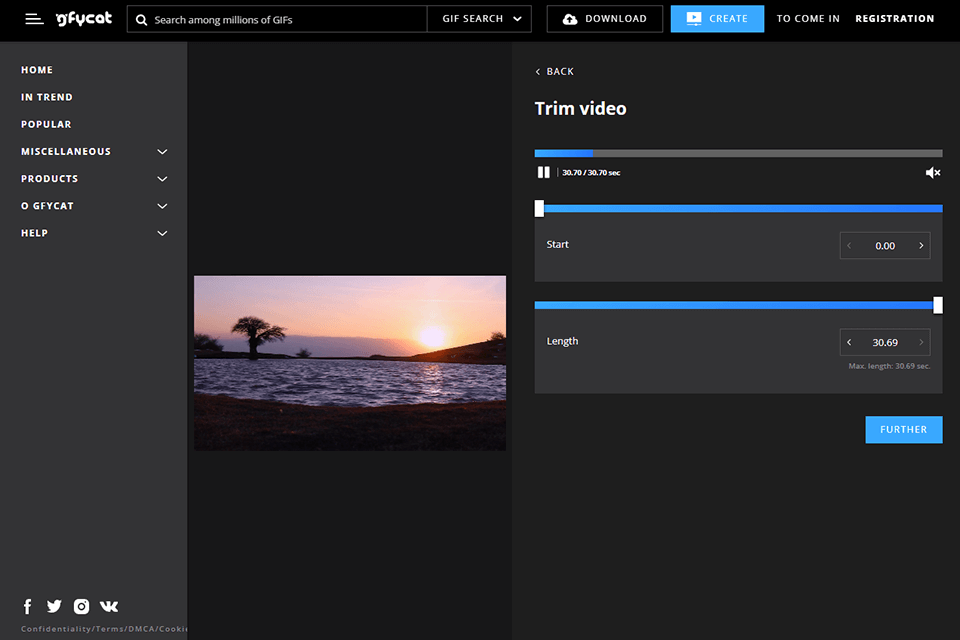A detailed caption of the image with multiple user interface elements:

The image is set against a black background and prominently features the Gfycat website interface. At the top, the Gfycat logo is displayed, accompanied by three navigation bars. There is a search bar to find GIFs, along with buttons labeled "GIF," "Search," "Download," and a blue rectangle labeled "Create." The interface also includes options for registration, which leads to the homepage displaying trending, popular, and miscellaneous products.

Below these elements, there is a section labeled "OGFYCAT" and "Help," indicating a return or support option. The video trimming interface is visible, showing a progress bar with a pause button and a speakerphone icon marked with an 'X,' indicating the mute function. This progress bar is partially filled and shaded to approximately 20% blue.

Another complete blue-shaded bar is present, indicating the start and total length of the video. The video length is marked as 30.69 seconds. There is also a blue rectangle with the text "Father" written in white. The background of the interface displays an image of the ocean, dotted with palm trees, blending seamlessly into the digital layout.